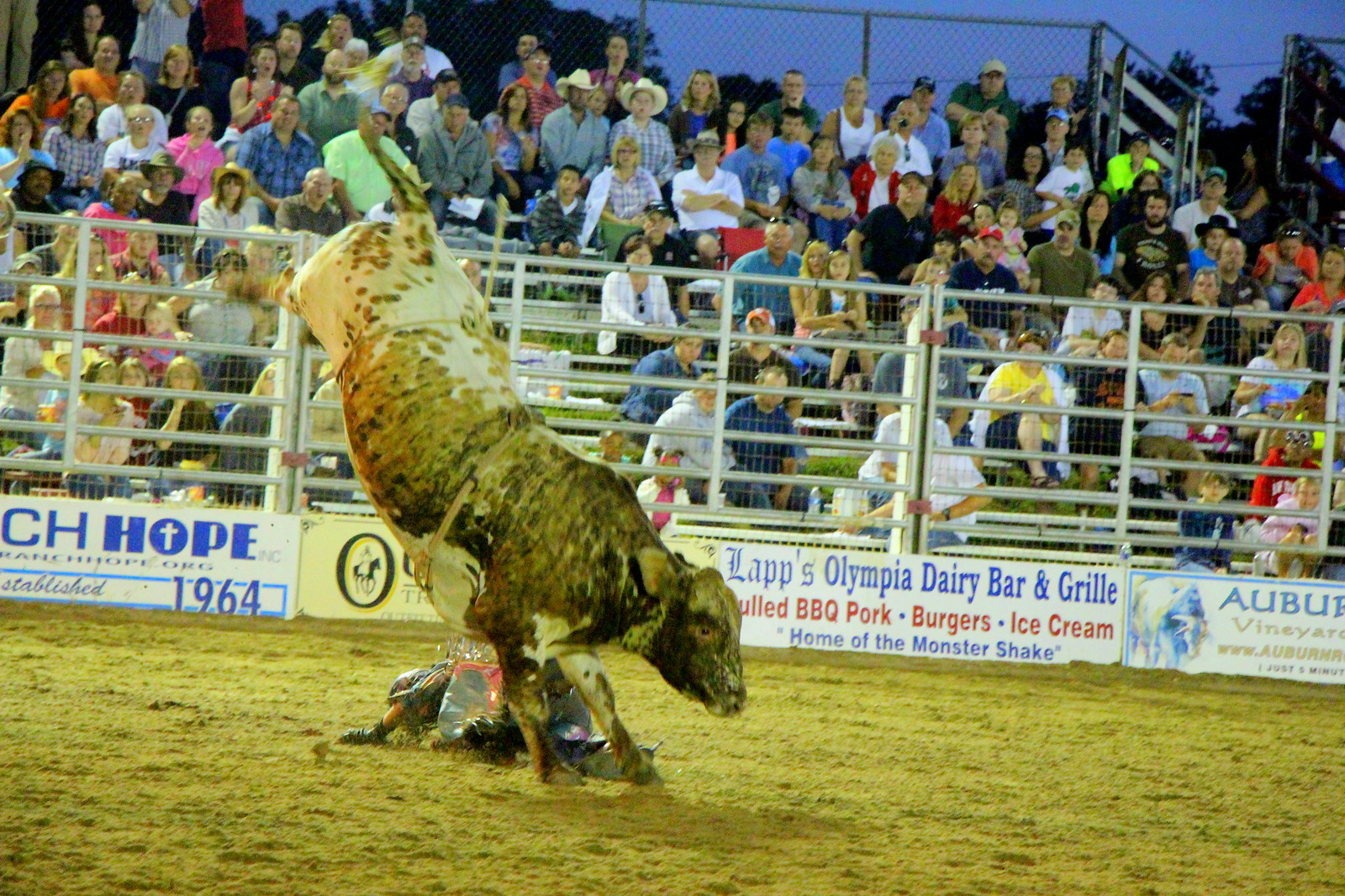This vibrant image captures the dramatic moment of a rodeo where a bull is seen mid-kick, its hind legs thrust high into the air as it throws off a cowboy. The bull, a striking mix of brown and white, has its front legs planted firmly on the ground and its head angled downwards, showcasing its power and agility. The cowboy, who appears to have been recently ejected, lies on the ground beside the bull in the dusty rodeo arena.

In the background, a dense row of trees frames the scene against a darkening blue sky, suggesting the event is taking place in the early evening, perhaps just before nightfall. The spectators seated on bleachers are a colorful mix, some wearing cowboy hats and others dressed in bright orange and pink attire. The crowd, numbering around 50 to 60 people, watches with anticipation and excitement.

A sturdy white fence separates the audience from the rodeo ring for safety, and various advertisements line the arena. Notable among them is a banner for "Laps Olympia Dairy Bar and Grill," promoting food items like pulled barbecue pork, burgers, ice cream, and the infamous Monster Shake. Another banner mentions "Auburn Vineyard," and there’s a partial sign that includes "CH Hope, Established 1964," hinting at perhaps a local establishment or sponsor.

The scene is illuminated by lights shining down on the arena, adding to the thrilling atmosphere of this classic rodeo moment.